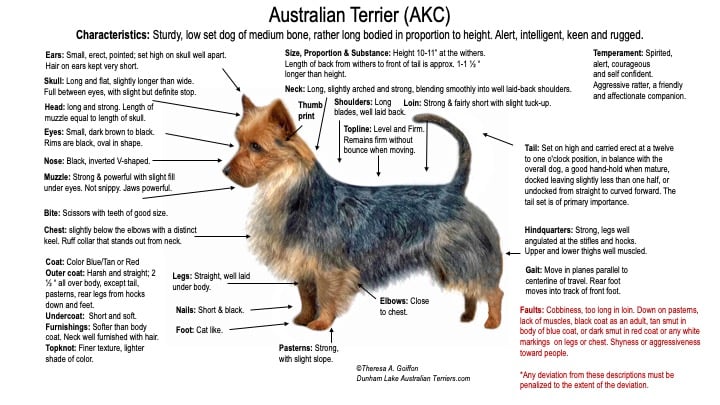This is an informative diagram of an Australian Terrier, designated by the AKC (American Kennel Club). Set against a white background with black and brown text, the illustration showcases a dog standing upright with its tail raised, head lifted, and ears perked. The diagram is densely annotated with arrows pointing to various parts of the dog's body, detailing its attributes.

At the top, the title "Australian Terrier" is flanked by "AKC." The diagram specifies the breed's characteristics: a sturdy, low-set dog with medium bone structure, a long body in proportion to its height, possessing an alert, intelligent, keen, and rugged demeanor. Each anatomical section such as the ears, skull, head, eyes, nose, muzzle, and bite is thoroughly described, including ideal sizes and proportions.

The diagram also identifies faults to be penalized, such as excessive length in the loin, adult black coat, and deviations from listed descriptions. Furthermore, there are sections detailing the coat, including both outer coat and undercoat, chest, hindquarters, elbows, and overall proportions, along with notes on temperament and height. The meticulous annotations provide a comprehensive guide, likely intended for judging purposes or breed standard education.